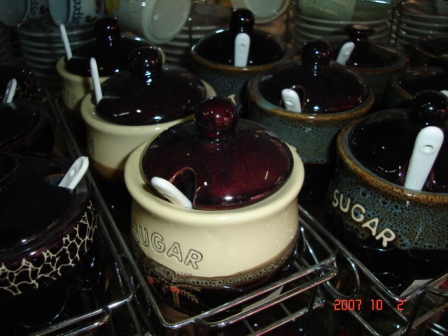The photograph showcases an array of colorful sugar jars, each nestled in small metal cages. The jars are organized by color: on the left, they are dark red; in the center, they are white; and on the right, they are green with black dots. All visible jars prominently display the word "SUGAR" in capital lettering. Each jar is equipped with a thick ceramic lid featuring a round knob, and a white measuring spoon protrudes from a cutout space in the lid. The scene is somewhat dimly lit, suggesting the use of a camera flash that doesn't fully illuminate the background, yet brings the foreground jars into clear focus. The arrangement is orderly, with three jars per metal cage, adding a touch of visual symmetry to the setup.